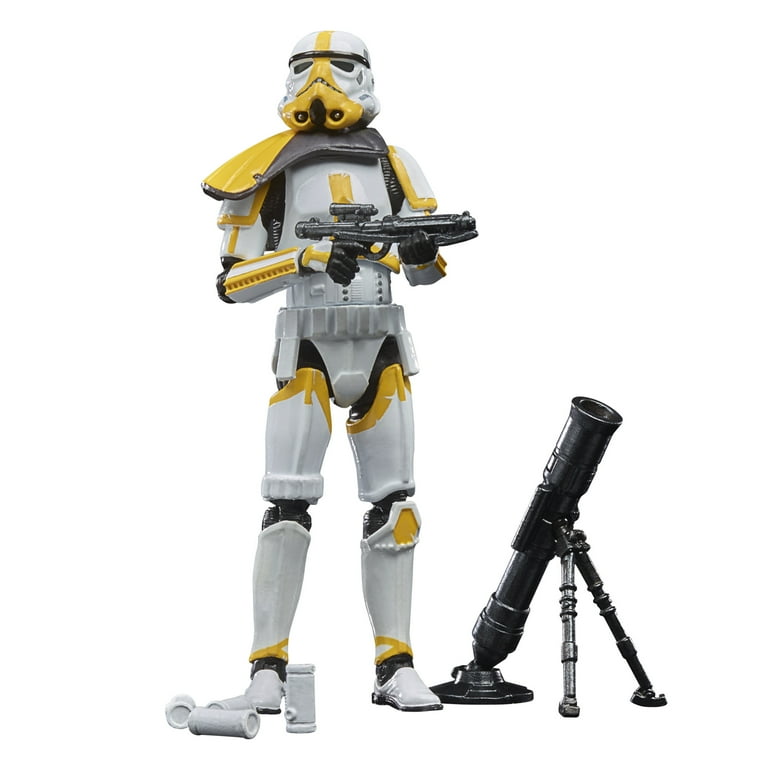The image depicts a detailed and highly realistic action figure of a Stormtrooper. This particular Stormtrooper is unique with distinctive yellow markings that suggest it might be a special forces variant, featuring a yellow stripe down the center of its helmet, a yellow line on its chest plate, and a yellow knee pad on one knee. The Stormtrooper is armed with a black rifle, and at its feet, there are four white canisters, likely intended to represent grenades or some sort of explosive devices. To the right of the Stormtrooper, a black, wide-barreled launcher, potentially a grenade or rocket launcher, stands on a bipod, made entirely of metal. The launcher, which can be adjusted for firing, adds a menacing touch to the scene. The overall composition of the photo highlights the impressive design and detail of the miniature figures and accessories.